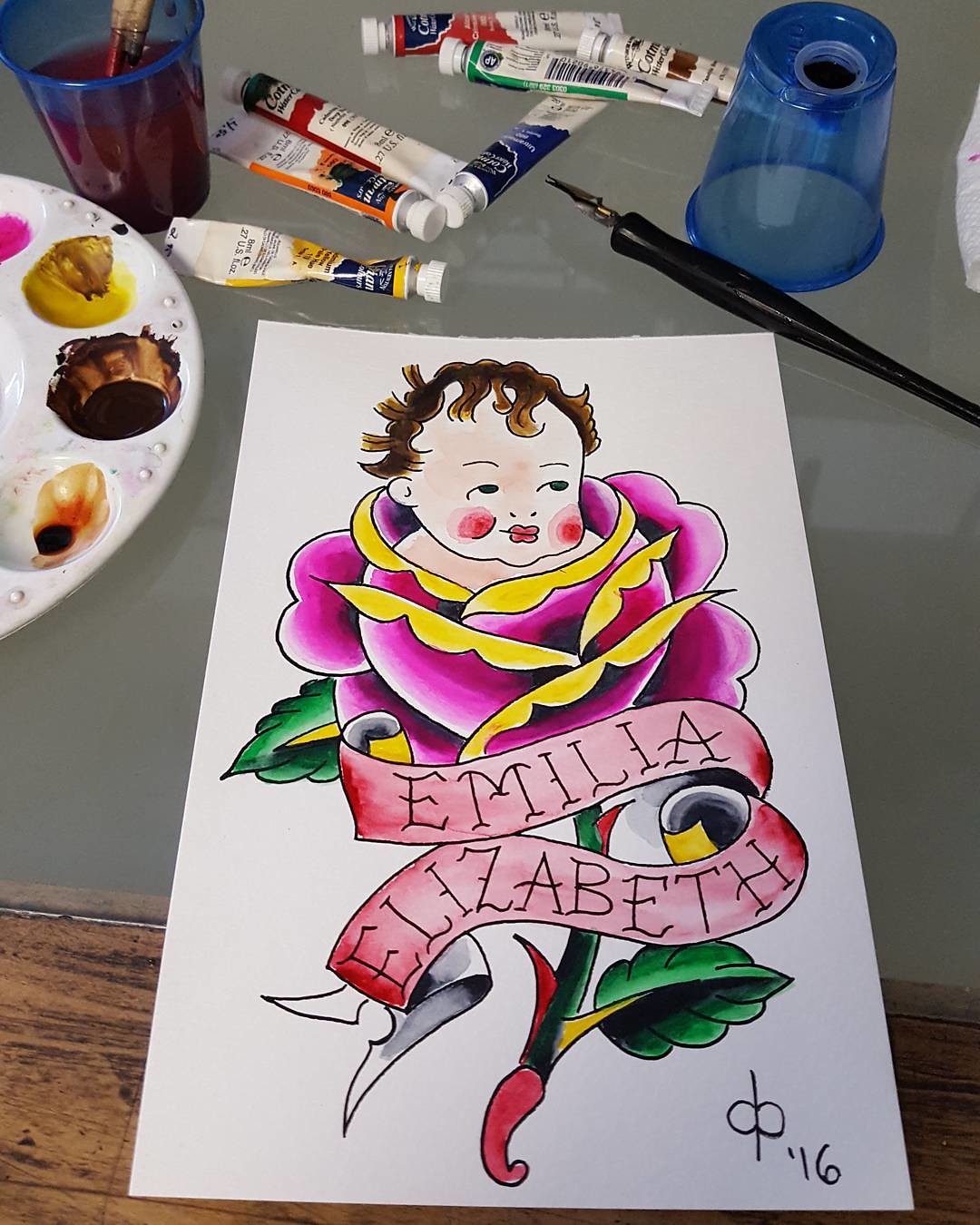This image captures a beautifully executed painting on a rectangular white sheet of paper. The artwork portrays a swaddled baby with rosy cheeks and brown hair, nestled within the petals of a pink and yellow rose. Below the serene scene, a banner elegantly displays the name "Amelia Elizabeth" in a complementary font. Surrounding the banner, vivid green and red accents add a touch of vibrancy to the composition. The sheet of paper rests on a table with a wooden frame and a glass center, providing a sturdy yet transparent surface. Arrayed above the painting are various painting supplies, including several small canisters of paint, paintbrushes, a cup of water, and a dish likely used for mixing colors. The overall scene exudes a sense of creativity and meticulous attention to detail.